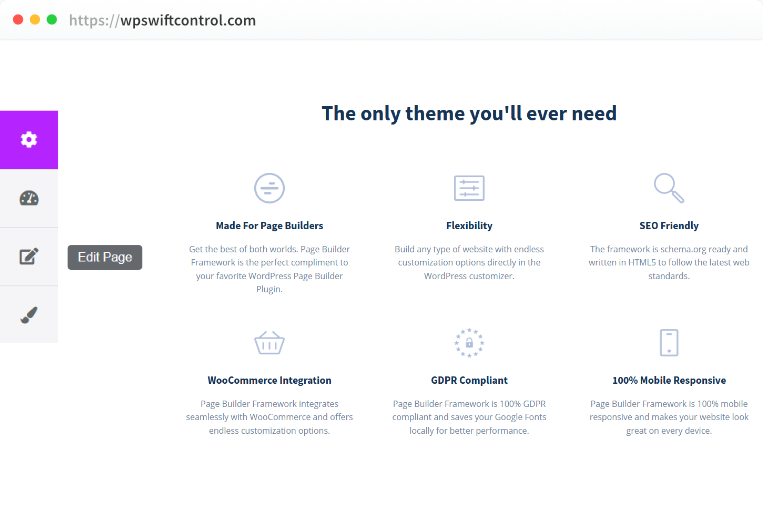This screenshot, captured on a MacBook, showcases a segment of the website wpswiftcontrol.com. The image features a clean, white background and highlights the tagline: "The Only Theme You'll Ever Need." Below this proclamation, six different key features are neatly listed: 

1. **Made for Page Builders** - Promoting the website as an excellent tool for constructing web pages.
2. **Flexible**
3. **SEO Friendly**
4. **100% Mobile Responsive**
5. **GDPR Compliant**
6. **WooCommerce Integration**

On the left side of the screen, there is an option for further page editing. Towards the bottom, there is a settings icon presented in a purple background box. Additionally, details about a settings automator with associated listings are displayed, suggesting customization and automation features for theme management.